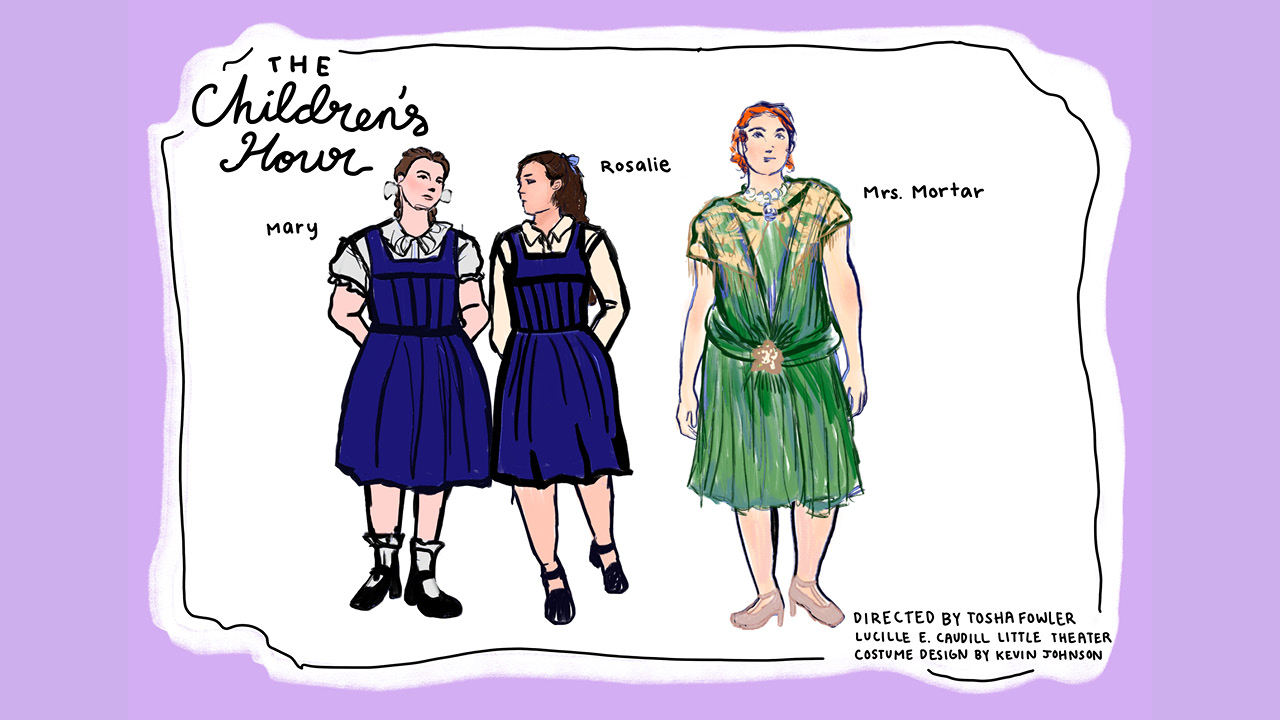This advertisement for "The Children's Hour," set against a light purple background, features a white rectangular frame with the title prominently displayed. Inside the frame, three women are drawn with careful detail. On the left, Mary wears a navy blue dress over a white blouse, accessorized with a blue hair tie and black Mary Jane shoes with light blue socks. Beside her, Rosalie donnes a similar outfit: a navy blue dress and white blouse, but she forgoes the socks, complementing her look with a darker blue bow in her hair and black Mary Janes. On the right stands Miss Mortar in a green dress with yellow detailing near the shoulders, a star-patterned belt, a white pearl necklace, and tan shoes. She has distinct orange hair. The illustration notes that the play is directed by Tasha Fowler, with costume design by Kevin Johnson, and is presented by the Little Theater.